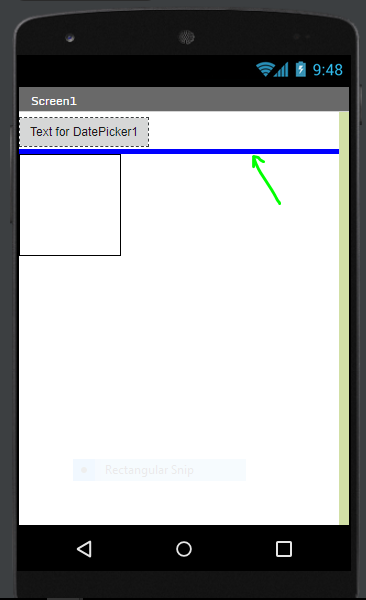This image showcases a tutorial on app design layout demonstrated on an iPhone. The screen displays a detailed design of an app page with several elements. At the top, there's a simple gray rectangular bar featuring the label "Screen One" in white, positioned in the upper left corner. Directly below this header, a gray rectangular box marked "Text for Data Picker One" serves as a possible subheader. 

A prominent dark blue horizontal line separates the subheader from the main content area. In the upper left section of the content area, there's a white box outlined in black. Directly beneath this box is another white field, currently void of any information.

Interestingly, an overlay of a neon green arrow points diagonally upward towards the blue horizontal line from the lower right direction, though it lacks any accompanying text or explanation. The screen also includes standard cell phone icons typically found in the status bar and navigation bar, with the time displayed as 9:48 in the upper right corner.

The overall design points to a minimalist approach with essential elements often used in app development tutorials, emphasizing clarity and structure. The absence of additional text or imagery keeps the focus on the layout elements, making this a clear example of instructional content for mobile app design.